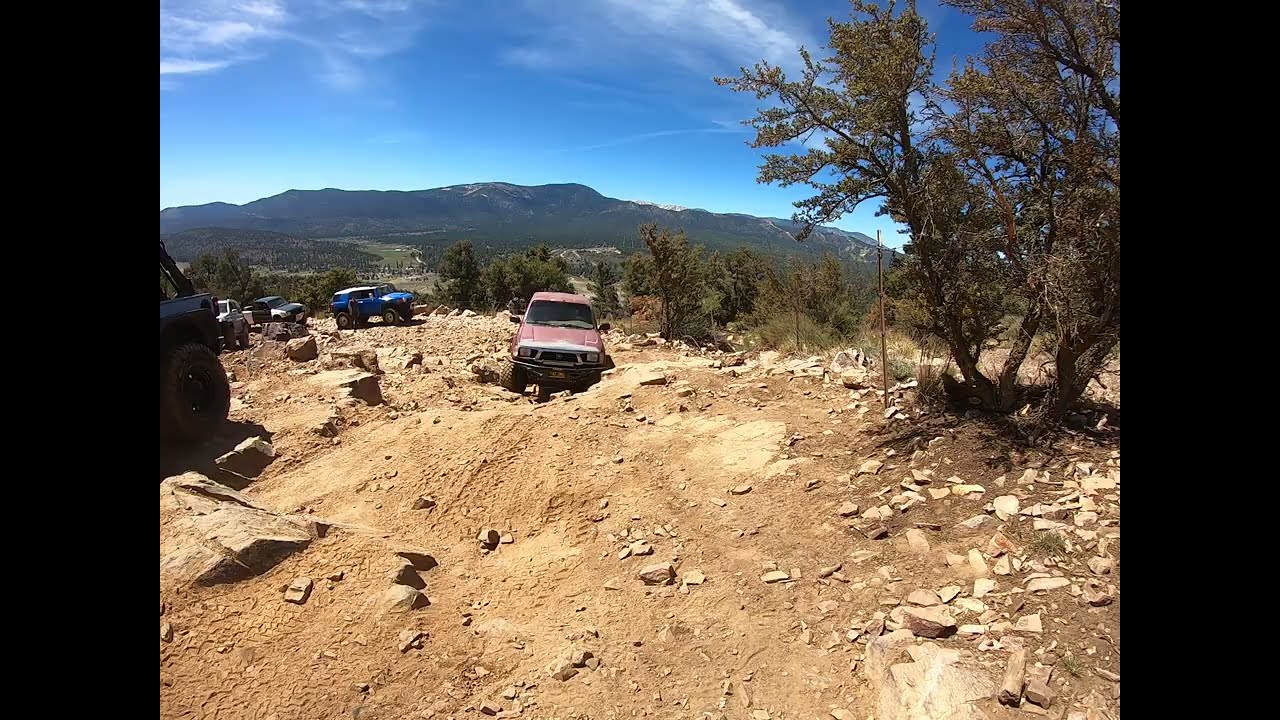The image depicts a rugged, outdoor scene set in a hilly, dirt area with a mountainous background. The sky above is a brilliant blue with wisps of feathery white clouds. The foreground features uneven, dusty brown terrain littered with small rocks and chunks of dirt. Central to the image is an older-looking red and white truck positioned with its front end facing the viewer. To its left, partially behind it, is a newer blue SUV, likely a Jeep or Hummer, sporting rugged off-roading tires. Further back, two additional SUVs with similar rugged tires can be seen, indicating the area is popular for off-road activities. A moderate-sized tree with green leaves stands in the upper right corner. Although the background is primarily mountainous and somewhat barren, trees sporadically populate the distant valleys, adding to the scene's isolated yet adventurous feel. This setting, bathed in the mid-day sun, conveys the atmosphere of an outdoor escapade in a Californian-like, dusty hill area.